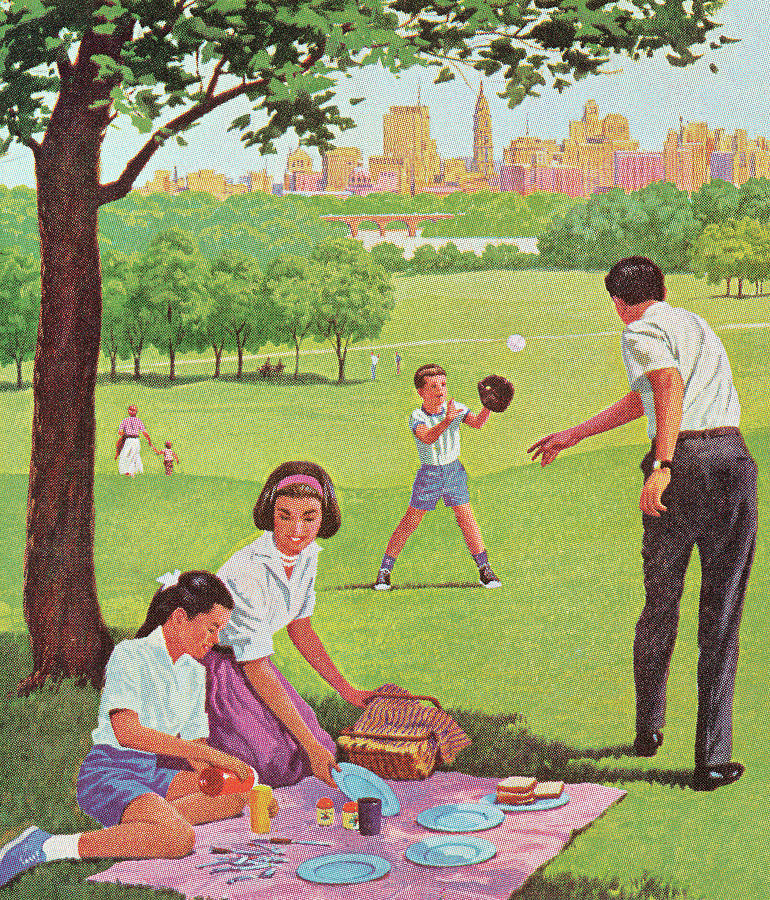The image is a detailed painting set in the 1940s or 1950s, depicting a family of four enjoying a picnic in a vast park with a cityscape, likely New York City, in the distance. Dominating the background are towering skyscrapers, reminiscent of the Empire State Building, along with a bridge spanning over a river. The park itself is expansive, with low-lying green lawns and scattered trees.

At the foreground of the painting, a pink picnic blanket is spread out on the grass. A young mother, characterized by her short brown bob, pink headband, pink skirt, and white blouse, is seated as she sets blue plates and silverware. She is arranging items from a brown picnic basket covered with a cloth. A plate with sandwiches is placed nearby. Her daughter, around 10 or 11 years old with dark brown hair tied with a white bow, is also wearing a white blouse paired with blue shorts and blue sneakers. The daughter is engaged in pouring a drink from a red cup into a yellow one, with silverware scattered at her feet.

To the right, the father and son are depicted in a game of catch. The father, dressed in a white short-sleeve shirt, black slacks, black dress shoes, and a brown belt, stands confidently as he throws a baseball. He has black hair and wears a wristwatch on his left hand. The son, with short blonde hair, wears a white striped shirt, blue shorts, blue socks, and black-and-white tennis shoes. He is poised to catch the incoming ball with his glove.

In the background, besides the striking urban skyline, multiple people are seen walking in the park, adding life to the serene and idyllic family scene. A tree on the left-hand side of the image provides additional framing and depth to this picturesque moment.